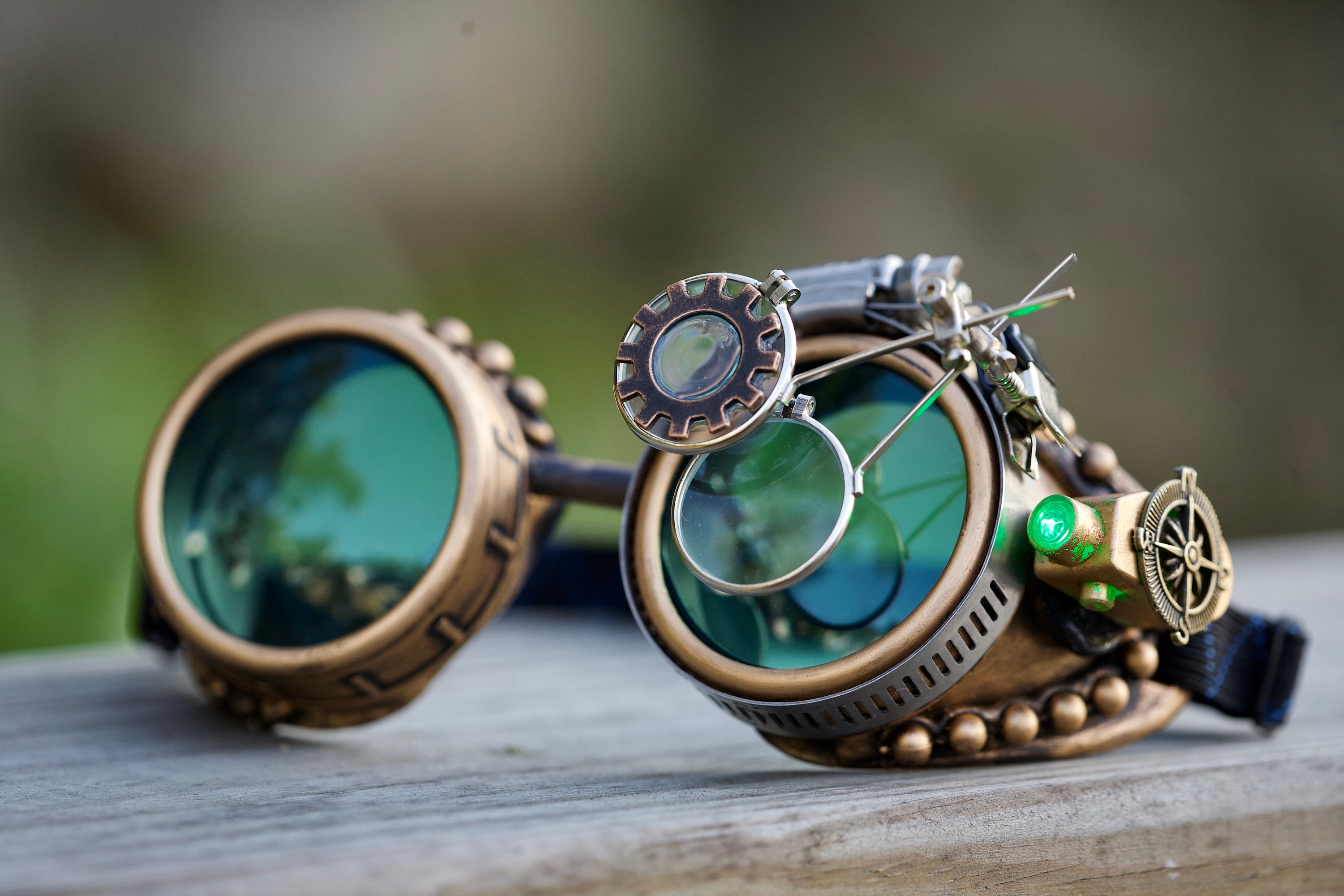These steampunk goggles are a fascinating piece of intricate craftsmanship, featuring a blend of classic and futuristic design elements. The main lenses are green, providing a distinctive tinted view. One of the key features on the left eyepiece includes two additional magnifying lenses that can slide over the main green lens for enhanced magnification; one of these is clear while the other is adorned with a gear, reminiscent of watchmaker tools. On the right side, the goggles have a metal rim and a compass rose attached to a vibrant green LED light, adding both functionality and aesthetic appeal. The golden-colored goggles are quite thick and appear to be constructed from sturdy materials, complemented by round spheres and ornate detailing along the edges and backside, which is fastened with a black strap. The image, which seems computer-generated, captures the goggles in sharp focus against a blurred backdrop of greens and grays, placed on a worn-down wooden table, reinforcing their vintage and industrial charm.